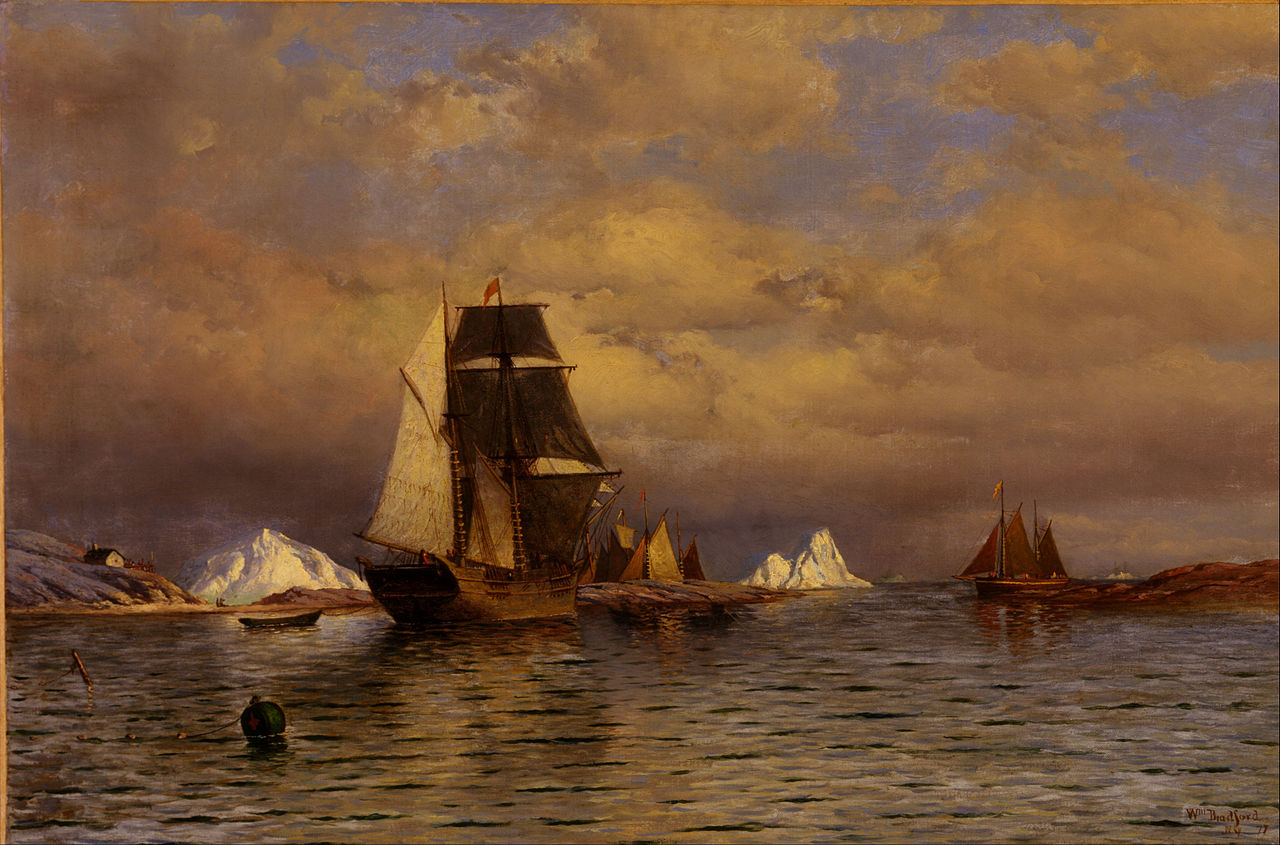This evocative painting, reminiscent of an old oil photograph, captures a dramatic maritime scene set against a foreboding, dark sky dominated by purplish, pinkish, and white clouds with sparse light blue patches. The turbulent, dark water roils with waves, setting an ominous tone. At the forefront, a round flotation device with an attached chain floats on the churning sea, its attachment point obscured. The painting features two prominent ancient wooden sailing ships, likely 18th-century schooners, seemingly on a collision course, hinting at a potential naval confrontation. Both ships have their sails fully deployed as they navigate the choppy waters. To the left of the composition, a smaller boat or dinghy can be seen near the shore, where a tiny house perches on a hill. The landscape also includes White Hill to the left and another in the distant background. On the right side of the painting, a patch of brown land juts out into the water, accompanied by another small sailboat. Adding to the complexity, tents are visible on the land behind the ships, further enriching the detailed and storied tableau.